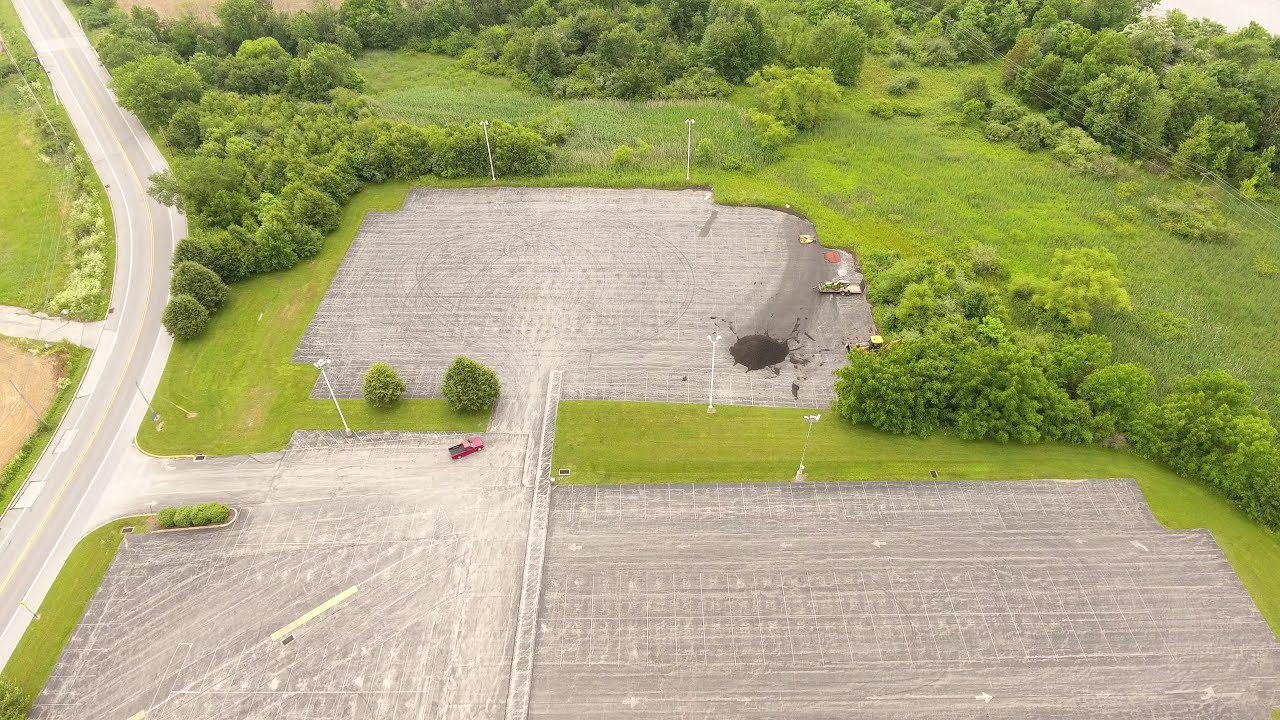This aerial photograph, likely taken by a drone or helicopter, offers a detailed bird's eye view of a countryside area. The top portion of the image features an expanse of trees, bushes, and grassy fields. Along the left edge, a road meanders from the top left corner, arches slightly inward towards the center, and winds down to the lower left corner of the image. To the right of this road lies a lush landscape of grassland and groves of trees.

In the middle part of the image, a distinctive gray cement area, resembling a paved parking lot, occupies the foreground. This main parking lot is large, almost rectangular but with rounded edges, and is nearly the width of the image. It is connected via a short path to another smaller parking area located directly above it. The large parking lot in the foreground contains a noticeable red car, while the smaller upper rectangle has a few indistinct vehicles. Overhead lights, presumably for illuminating the parking areas, are also visible within these cement sections.

The backdrop of the image is a verdant field dotted with multiple clusters of trees, providing a sharp contrast to the structured paved areas. Overall, the composition showcases a balanced blend of natural and man-made elements, perfectly capturing the tranquil rural setting.